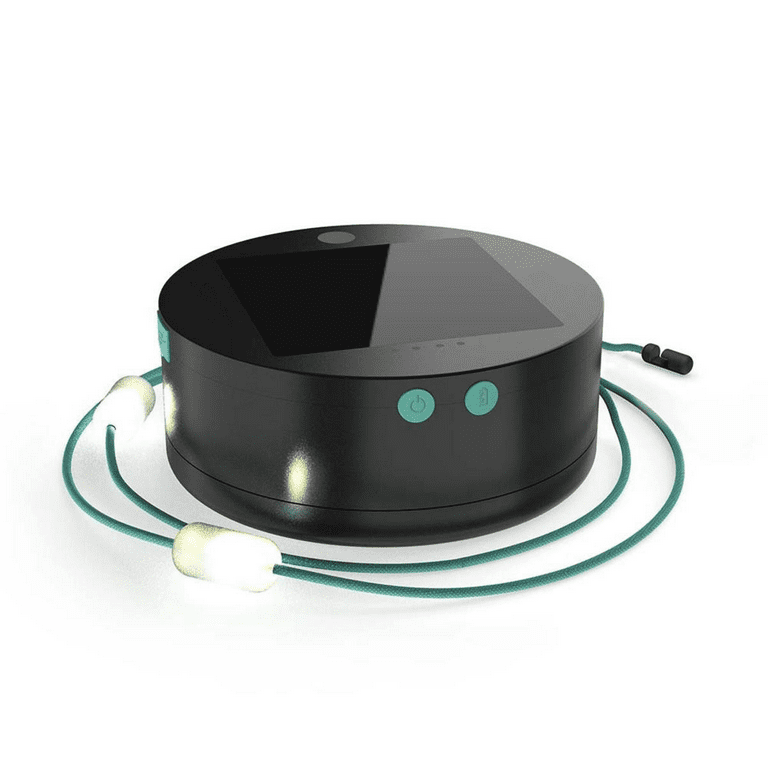This image depicts a sleek, black electronic gadget resembling a short cylinder or disc, reminiscent of an Amazon Echo Dot. The device features a shiny, rectangular screen on its top surface, possibly a display. It has two buttons on the front: a power button on the left and another, likely an indicator or function button, on the right. Both buttons are colored green. A cyan-colored cord, potentially a USB cable, is wrapped several times around the device. This cord has three distinct attachments: two white, puffy objects that resemble marshmallows, and a small black item at the end, possibly a microphone or connector. The entire setup is presented against a clean, white background, giving it a computer-generated appearance.